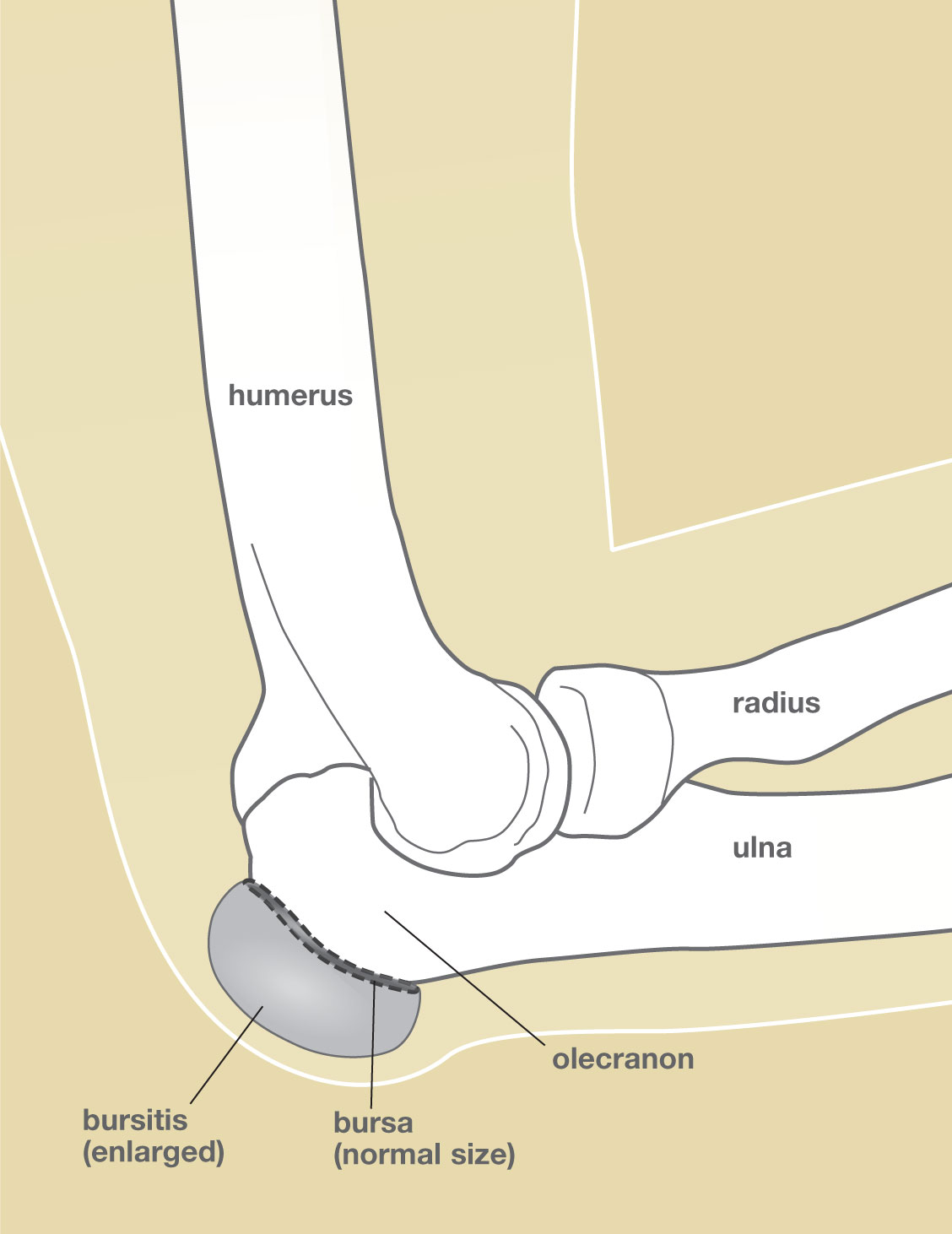The image is a detailed anatomical drawing depicting bursitis of the elbow. The background is a creamy brown, with the central figures outlined in white to resemble an X-ray view. The top bone, labeled as the humerus, is vertical, while the radius and ulna, which are horizontal, form the forearm. At the intersection of the humerus and ulna is a small black structure labeled as a bursa, indicating its normal size. A gray, enlarged representation of this bursa signifies bursitis—a condition characterized by inflammation of the bursa. The area around the affected bursa is also labeled as the olecranon. The bones and soft tissues are clearly delineated to emphasize their anatomical relationships and the swelling caused by bursitis.